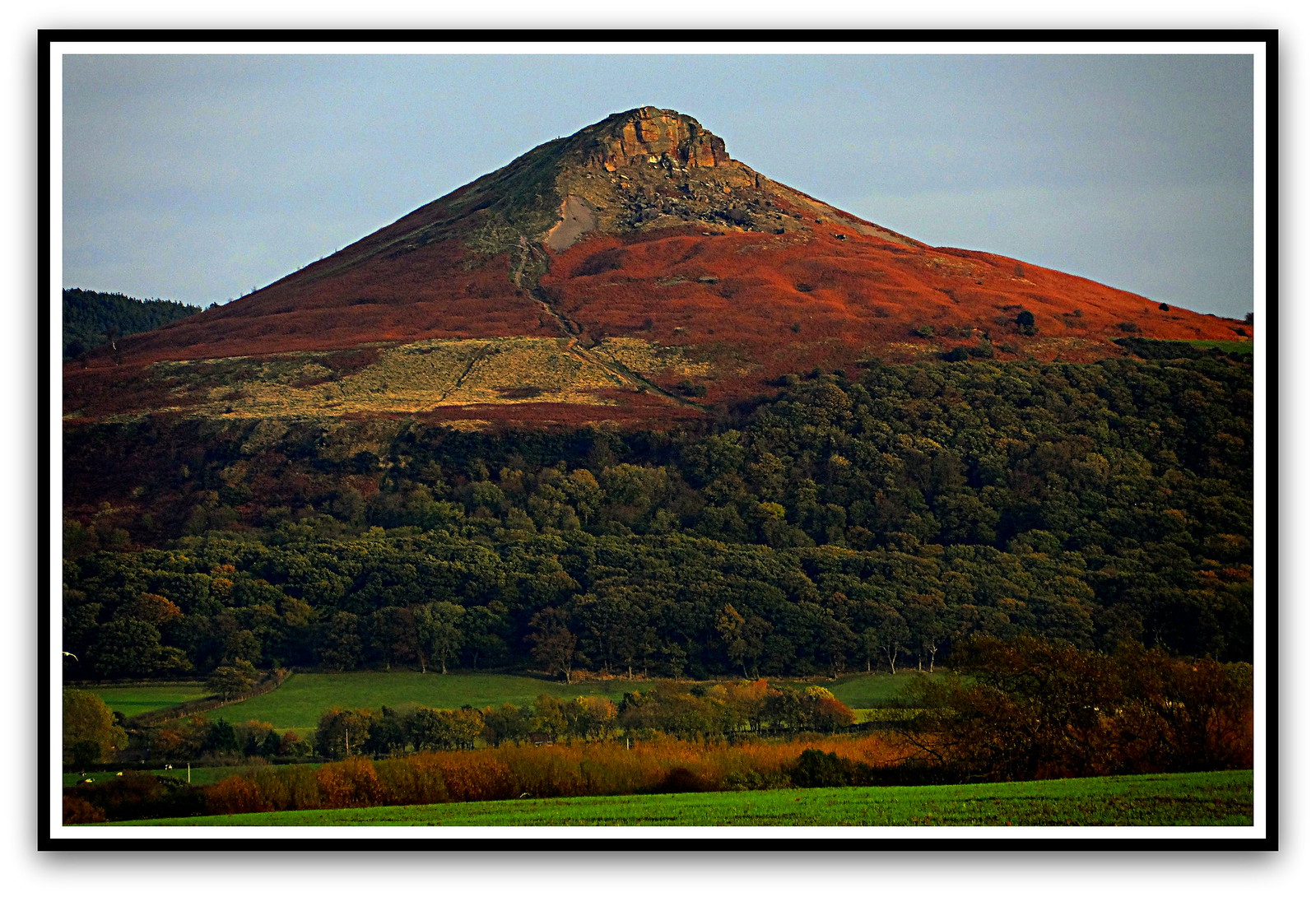This is a rich, postcard-like photograph, framed with a white and black border, depicting a captivating nature scene dominated by a prominent mountain. The mountain spans the width of the horizontally rectangular image, transitioning from a craggy, rocky peak at the top down to a vibrant midsection adorned with bright red-orange formations or possibly foliage in full autumn bloom. Lower down, the mountain's base merges into a thick, dark green forest, which extends in a dense grove. Just before this forest, the left side features patches of yellow flowers. The scene further transitions to a manicured field of green grass, interspersed with brown and yellow bushes, suggesting a later stage of autumn. Multiple layers of greenery and natural textures create a harmonious blend from the bottom to the mountain peak. Finally, the mountain and its surrounding landscape are set against a backdrop of a clear blue sky, enhancing the overall allure of the image.